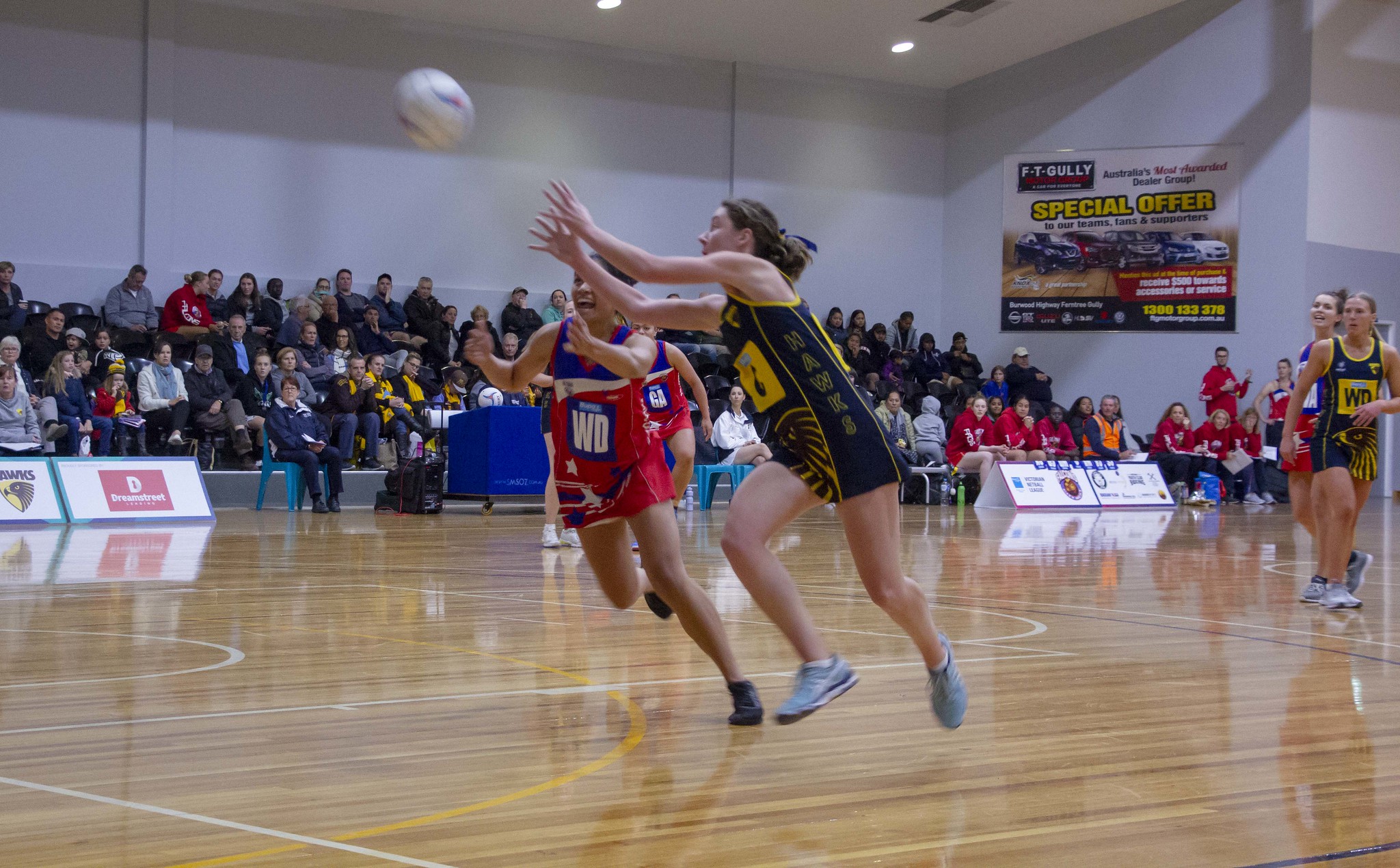The photograph captures an indoor girls' basketball game taking place in a high school gymnasium. The setting features a relatively small crowd seated in the stands, attentively watching the game. The image prominently displays six players: one team is sporting red and blue uniforms, while the opposing team is dressed in blue and yellow. At the center of the action, one player in a blue and yellow uniform is seen reaching up as if to catch a ball, which resembles a volleyball despite the basketball court setting. The high-gloss wooden floor of the court reflects the players, emphasizing the dynamic movement of the game. Surrounding the court are various advertisements, including a poster with the text "PT Gully," an indication of a special offer, and images of trucks. The gymnasium itself features gray walls, a white ceiling with overhead lighting, and additional players can be seen seated on the sidelines, ready to participate in the game.